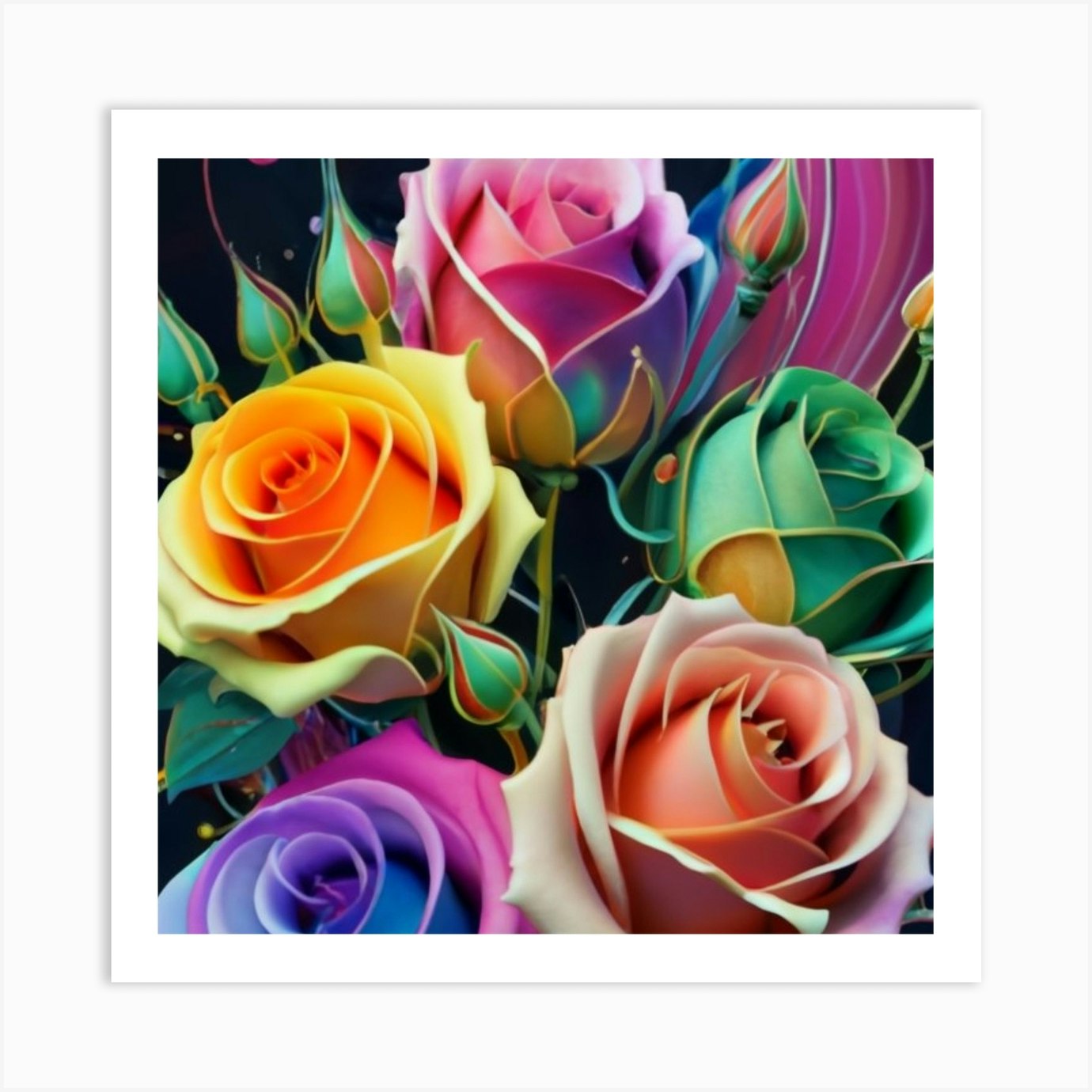The image is a vividly detailed, fantasy-style painting of a variety of colorful roses and buds arranged in a square frame. The frame consists of a white border accented with a stark black line, emphasizing the vibrant display within. Central to the composition, on the middle left side, a yellow rose tinged with orange petals draws the eye, while to its right, a striking teal-colored rose offers a contrasting cool hue. Above these, positioned at the top middle, blooms a delicate pink rose. Other prominent flowers include a peach-colored rose on the lower right and the partial view of a blue and pink rose on the bottom left. Scattered throughout are approximately six unopened buds, adding to the rich texture of the arrangement. The dark blue background enhances the brightness and softness of the colorful flowers, giving the painting a soft, harmonious feel.